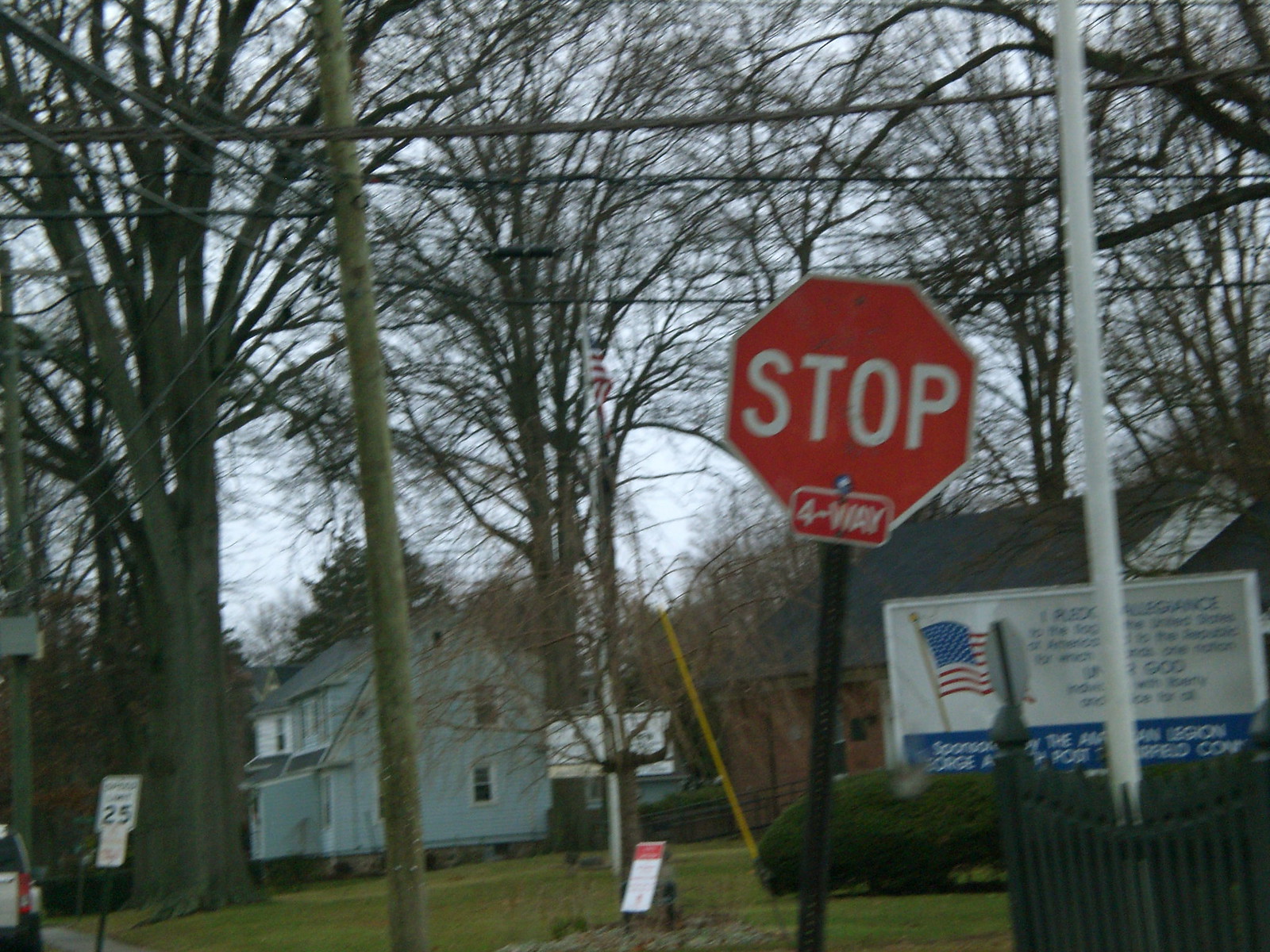This photograph, taken on a gray winter afternoon in a northern U.S. neighborhood, captures a four-way stop area framed by leafless trees under a white sky. To the left, there's a blue two-story house with part of a car visible nearby. A brick building stands to the right, mostly obscured by a sign displaying the Pledge of Allegiance and an American flag. A prominent feature is the stop sign with a "four-way" marker and a speed limit sign indicating 25 miles per hour. The ground is covered in sparse, grassy patches, and there's a black iron fence in the bottom right corner. The image has a hazy or blurry quality, adding to the wintry atmosphere. Electrical poles and a small set of green bushes are also visible, contributing to the suburban setting.